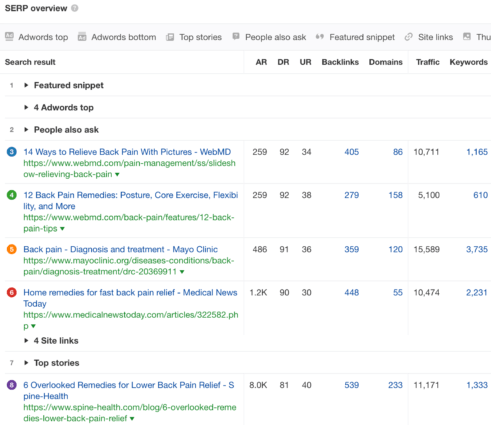This is a highly detailed screenshot from a computer or laptop monitor showing the backend interface of the AdWords program. The image features various statistics and active links, with the top-left corner prominently displaying "SERP Overview" in bold black text.

Below this heading, a series of labels appears in gray: “AdWords top,” “AdWords bottom,” “top stories,” “people also ask,” “featured snippet,” and “site links.” Next to these labels is a calendar icon with "THU" written in bold black text to its right.

Underneath this section, "Search Result" is clearly marked, followed by a labeled section starting with "1," which includes a rightward black triangle arrow indicating a "featured snippet." Beneath this is another similar arrow next to "AdWords top." The next line is labeled "2," also with a right triangle arrow pointing to "people also ask."

On the right side, there are labels in bold black text for metrics such as AR, DR, UR, backlinks, domains, traffic, and keywords, though this section appears empty.

Moving down, there is a series of links highlighted in blue, each accompanied by green URLs beneath. To the left of these links are various colored icons (blue, green, orange, red, and purple). Some of the links include:
1. “14 ways to relieve back pain with pictures” - WebMD
2. “12 back pain remedies: posture, core exercises, flexibility, and more”
3. “Back pain diagnosis and treatment” - Mayo Clinic
4. “Home remedies for fast back pain relief” - Medical News Today

Additionally, under the "Top Stories" heading in bold black text, a blue link reads "Six overlooked remedies for lower back pain relief" by Spine Health, listed next to a purple icon.

Metrics such as AR, DR, UR, backlinks, domains, traffic, and keywords are displayed here, with varying numbers in both blue (hyperlinked) and black text.